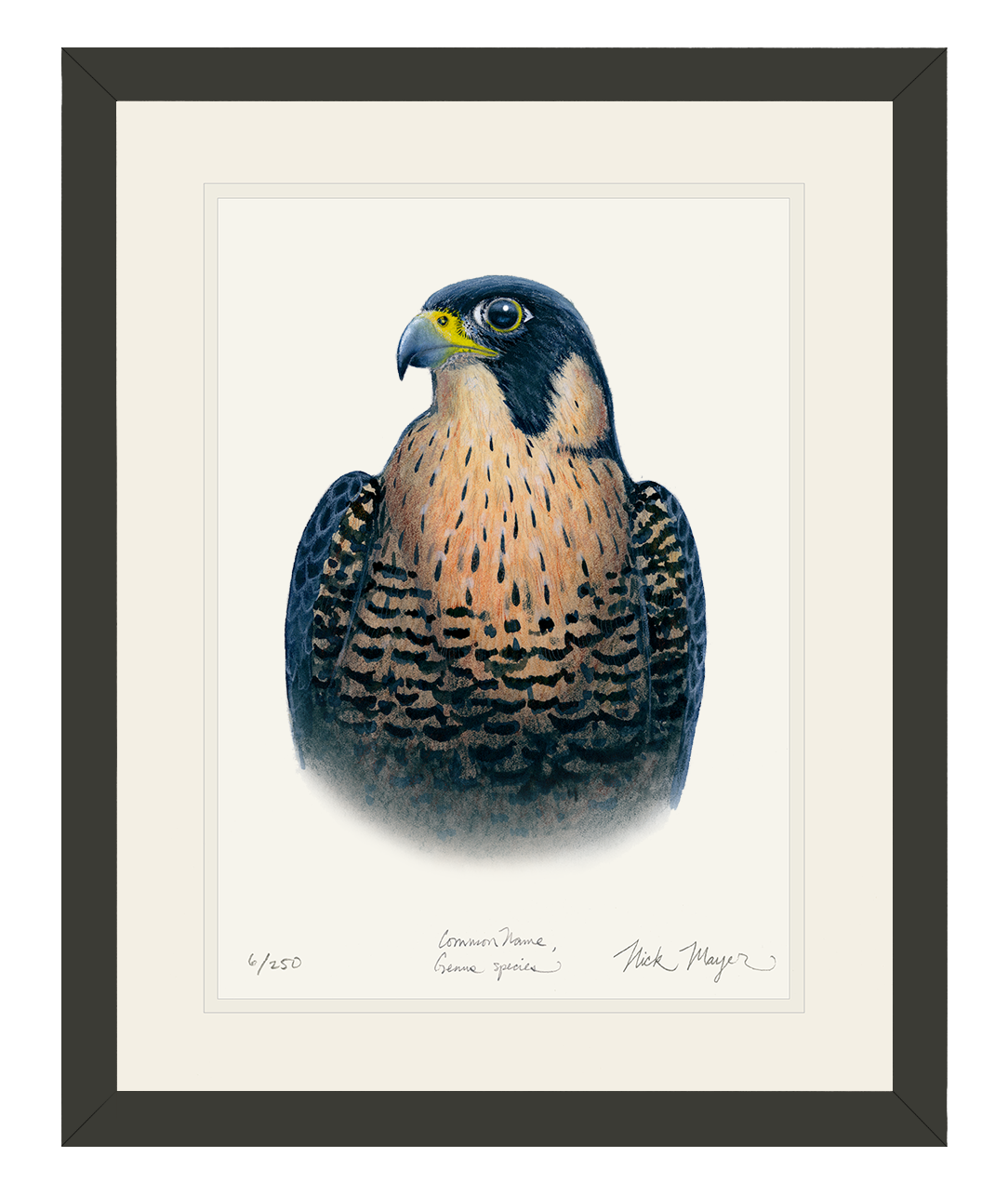The image is a detailed hand-drawn artwork depicting a falcon viewed from the front. The falcon's head is tilted to the side, showcasing one eye looking directly outward. Its short, curved beak is gray with yellow at the nostril, adding to the realistic portrayal. The bird's head is mostly black, while its neck features a blend of orange and black. The chest and wings are similarly patterned with black and orange speckles, displaying a striking contrast. The falcon's dark, hooded head and speckled orange wings contribute to its majestic appearance. The artwork features no background color, accentuating the bird against a white backdrop. At the bottom of the picture, it is labeled "6/250," indicating its limited edition status. There are words written, including "common name genus species," which appear to be part of a labeling template. The artist, Nick Meyer, has signed the piece. The artwork is framed with a double frame, comprising a light whitish-gray inner frame and a black outer frame, further emphasizing the bird's vibrant colors and intricate details.